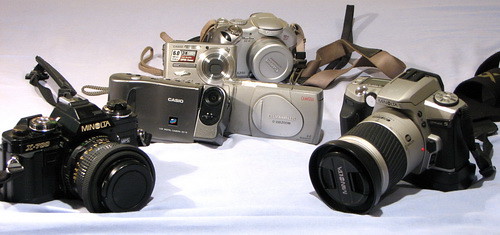The image is a color photograph showcasing an array of various cameras, meticulously arranged against a seamless white fabric backdrop that drapes from the surface they rest on up the wall. At the forefront, a black Minolta DSLR camera takes center stage, notable for its detachable zoom lens, adjustable from the front, and gold lettering that reads "Minolta." Positioned diagonally towards the right, it faces a silvery Minolta camera on the right side of the image, equipped with an extended lens and aimed towards the left center. Between these two prominent cameras sits a cluster of four compact point-and-shoot models, all in silver-gray. These smaller cameras, resembling tiny radios, include brands such as Casio and Canon, with two on the bottom supporting two more stacked on top. Additionally, an unidentifiable larger camera with a gray body and obscured branding is placed in the front center, sporting a black lens cover. A few camera straps are visible, adding to the scene of organized yet varied photographic equipment.